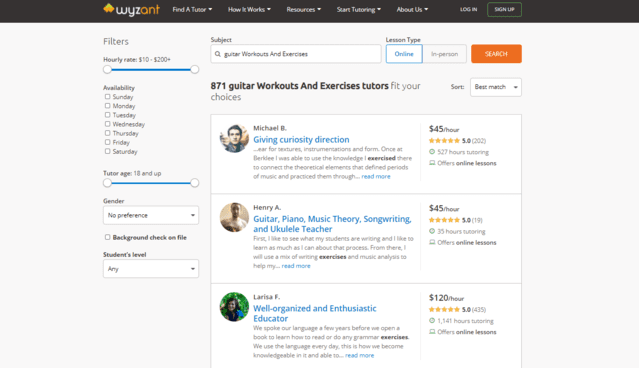The image showcases the homepage of the WISAMP website. Positioned towards the upper-left center, the site header prominently features the title "WISAMP." Adjacent to it is a navigation menu including the options: "Find a Tutor" with a drop-down arrow, "How It Works" with a drop-down arrow, "Resources" with a drop-down arrow, "Start Tutoring" also with a drop-down arrow, and "About Us" with a drop-down arrow. To the far right of the menu, there are buttons labeled "Log In" and "Sign Up."

Beneath the header, a filter section is present, starting with an "Hourly Rate" filter, which ranges from $10 to $200+ and features a blue slider bar with adjustable circular knobs on both ends. The next filter is "Availability," accompanied by checkboxes for each day of the week. Following this is the "Tutor Age" filter, similar in design to the hourly rate slider. The "Gender" filter includes a box displaying the option "No Preference" with a drop-down arrow.

Further down, there are additional filters for "Background Check" and "Student's Level." 

Central to the page are three sections showcasing individual tutors, each featuring profile pictures, star ratings, and hourly rates.